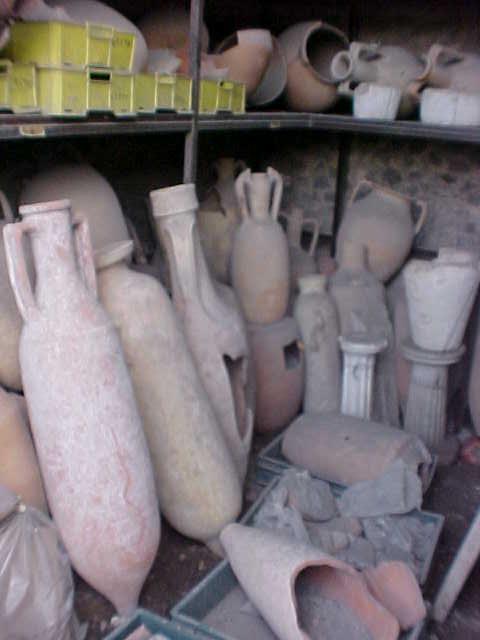The photo captures a pottery studio or storage area, likely for archaeological finds, showcasing a collection of ancient amphorae and other clay pots. The scene features a single black shelf at the top of the image, housing various clay pots and vases in shades of terracotta, white, pale gray, and neutral tan. Some are intact, while others are visibly broken or chipped. Yellow trays on the shelf hold shards and smaller pieces of pottery.

Below the shelf, a variety of amphorae and pots are arranged. There are approximately twelve pots on the ground, both broken and whole, leaning against each other and against two cast pillars. This area also includes four green trays filled with fragments and broken pottery parts. Some pots are grayish in color, and others exhibit unique features like windows cut out of them.

To the left, several intact amphorae are neatly lined up. These amphorae showcase characteristic ancient Greek designs, with small, skinny necks, rounded openings, and protruding handles that merge into the oblong bodies ending in pointed bases. A mix of small white and gray pedestals elevate some of the pottery, adding to the organized yet cluttered aesthetic of the studio. All items present vary in condition, with a notable number showing signs of damage.